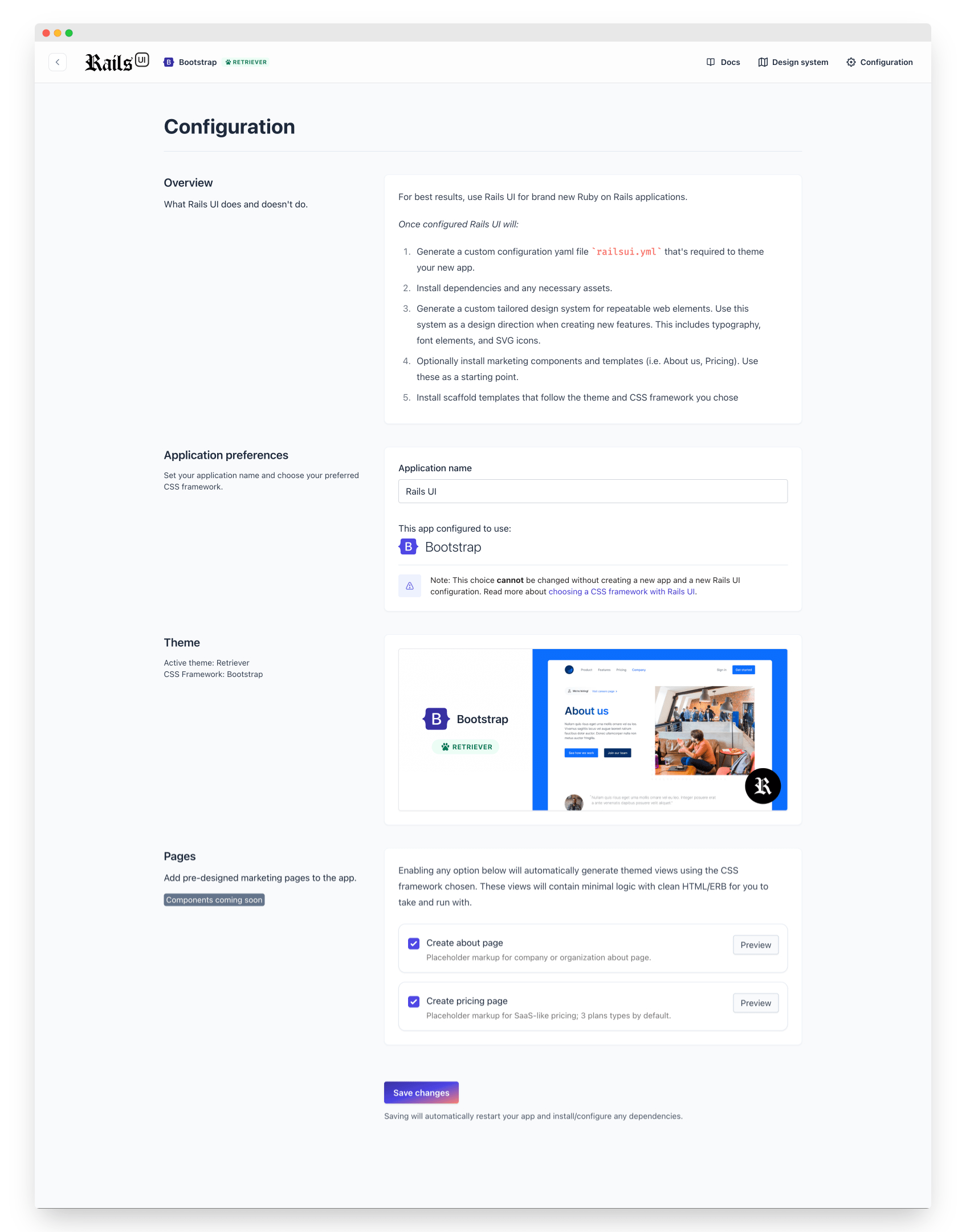The image features a distorted computer webpage that is difficult to read. At the top, there is a light gray bar containing the typical red, gold, and green circles found on browser windows. Below this, a large, bold black text box in light gray provides an overview of application processes and themes. The text is intentionally scrambled and incomplete, making it challenging to decipher.

Under the "Theme" section, a prominent blue box with a white interior reads "About Us." There is also a photograph of a shirtless man sitting on a couch. Below this, the section titled "Pages" features two drop-down menus, although their content is also heavily distorted and unreadable. At the bottom of the page, there is a "Subscribe" section, containing a centrally placed purple box with an orange side.